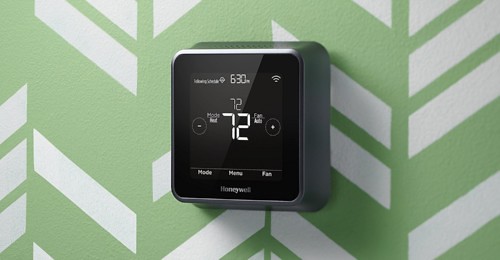The image is a carefully composed, landscape-oriented photograph featuring a thermostat as its central focus. The background is a soothing light mint green color, adorned with diagonally placed, rectangular white boxes that create a dynamic, arrow-like pattern on the wall. The thermostat itself, prominently positioned in the center, boasts a sleek, square design with a metallic steel shading.

The inner square of the thermostat is black, framing a subdued gray LED screen. At the top of the screen, the display shows the time "6:30 PM" along with a full Wi-Fi signal bar in the top right corner, indicating strong connectivity. Dominating the middle of the screen, a small numeral "72" is displayed above a larger "72," both in white, which likely represent the current and set temperatures respectively.

To the left of these numbers, the word "Modes" is displayed beside a circle with a minus sign, while on the right side, another circle with a plus sign appears. At the very bottom of the screen, in gray text, the options "Mode," "Memo," and "Fan" are listed from left to right. Below the black screen, the brand "Honeywell" is subtly inscribed, adding a touch of brand recognition to the sophisticated design.